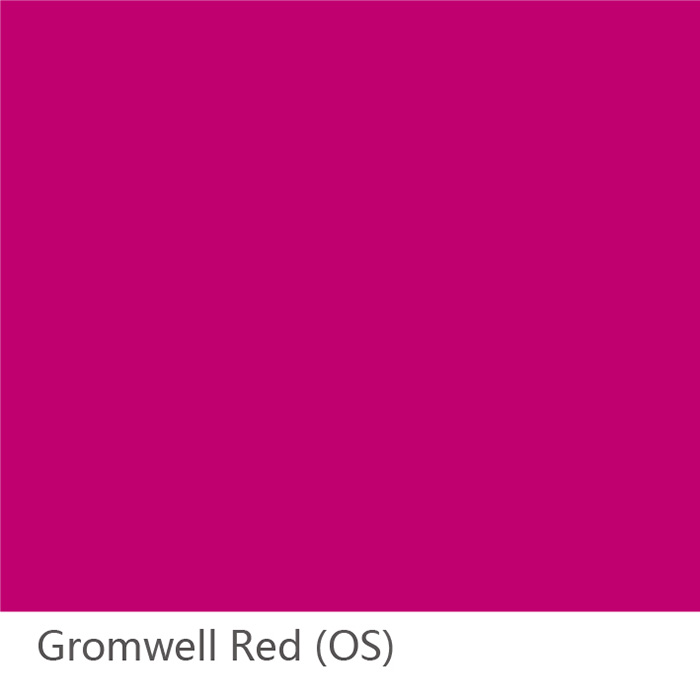The image depicts a vibrant violet square, which gradually transitions into a darker purple hue towards its top and edges, against a white background. The square, bearing a fuchsia-tinted purple, lacks any internal images or text, maintaining a solid color. Directly beneath the square is a white banner featuring the text "Gromwell Red (OS)" in dark gray, with the text aligned to the left side. This detailed layout suggests that the color of the square is named "Gromwell Red (OS)," possibly indicating a paint or color chip sample.